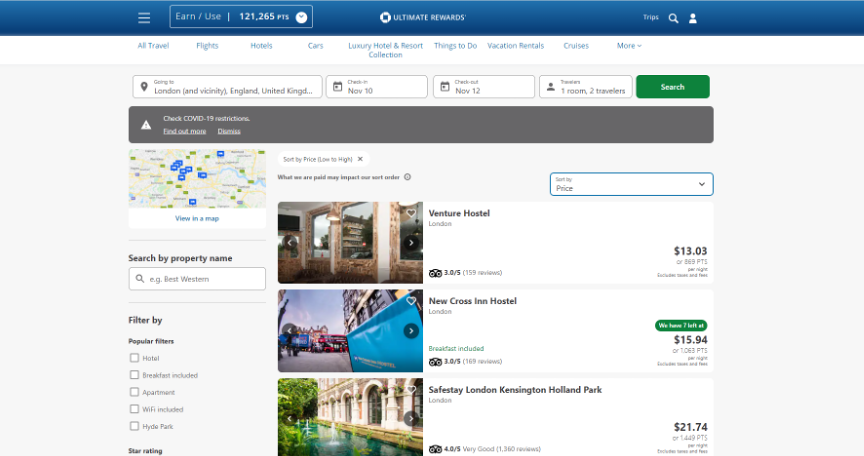In this detailed screenshot from a website, the top center prominently features the Chase Bank logo with the label "Ultimate Rewards." Adjacent to this, near the top right corner, there are options labeled "Trips" with a search symbol button and a profile button. Directly beneath this section, there is a series of interactive tabs for various travel-related categories, including "All Travel," "Flights," "Hotels," "Cars," "Luxury Hotel and Resort Collection," "Things to Do," "Vacation Rentals," "Cruises," and "More."

The main content area is organized into several text boxes for search parameters. The first text box on the far left, labeled "Going To," has been filled in with "London and vicinity, England, United Kingdom." The subsequent text boxes display selected dates: "Check-in" set for November 10th and "Check-out" for November 12th. The last text box indicates "Travelers," showing one room booked for two travelers. To the right of these input fields, there is a prominent green search button.

Below these search parameters, the results display three accommodation options: Venture Hostel, New Cross Inn Hostel, and Safestay London Kensington Holland Park. Each accommodation listing includes a thumbnail photo of the location on the left side, enhancing the visual appeal and ease of identification.